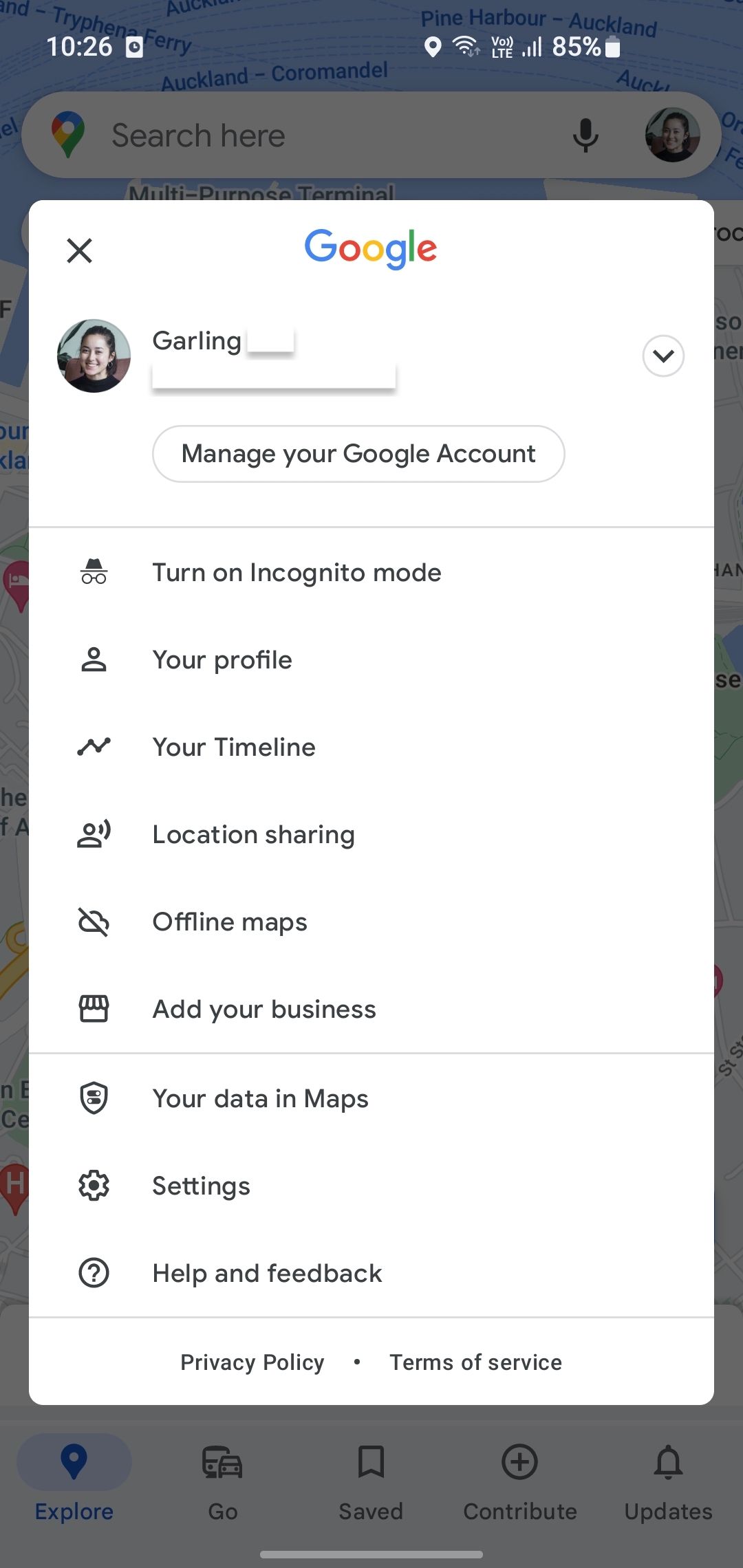In this image, we are presented with a screenshot taken from someone's phone, specifically displaying the Google app. The top right corner of the image shows a vertical battery icon, nearly full, depicted in white, with the battery percentage reading 85% next to it. Moving left, we encounter a fully-strengthened phone signal icon, followed by the acronym "VOLTE" also in white. To its immediate left, a fully-powered Wi-Fi signal icon is displayed, with a location pin icon just to the left of it. On the top left of the screenshot, the current time recorded is 10:26.

Dominating the central portion of the image is a pop-up box against a white background, labeled "Google" at its top center. On the far left of the pop-up is an 'X' symbol. Just below this header, there is a profile picture of a smiling woman. Adjacent to her image, the name "Garling" appears, with the following text obscured. Beneath this, the text "Manage your Google Account" is prominently shown.

Further down, the pop-up offers multiple settings options, including "Turn on Incognito Mode," "Your Profile," "Your Timeline," and "Location Sharing." The overall layout and user interface elements are typical of the Google app, providing a concise overview of the account management features available to the user.